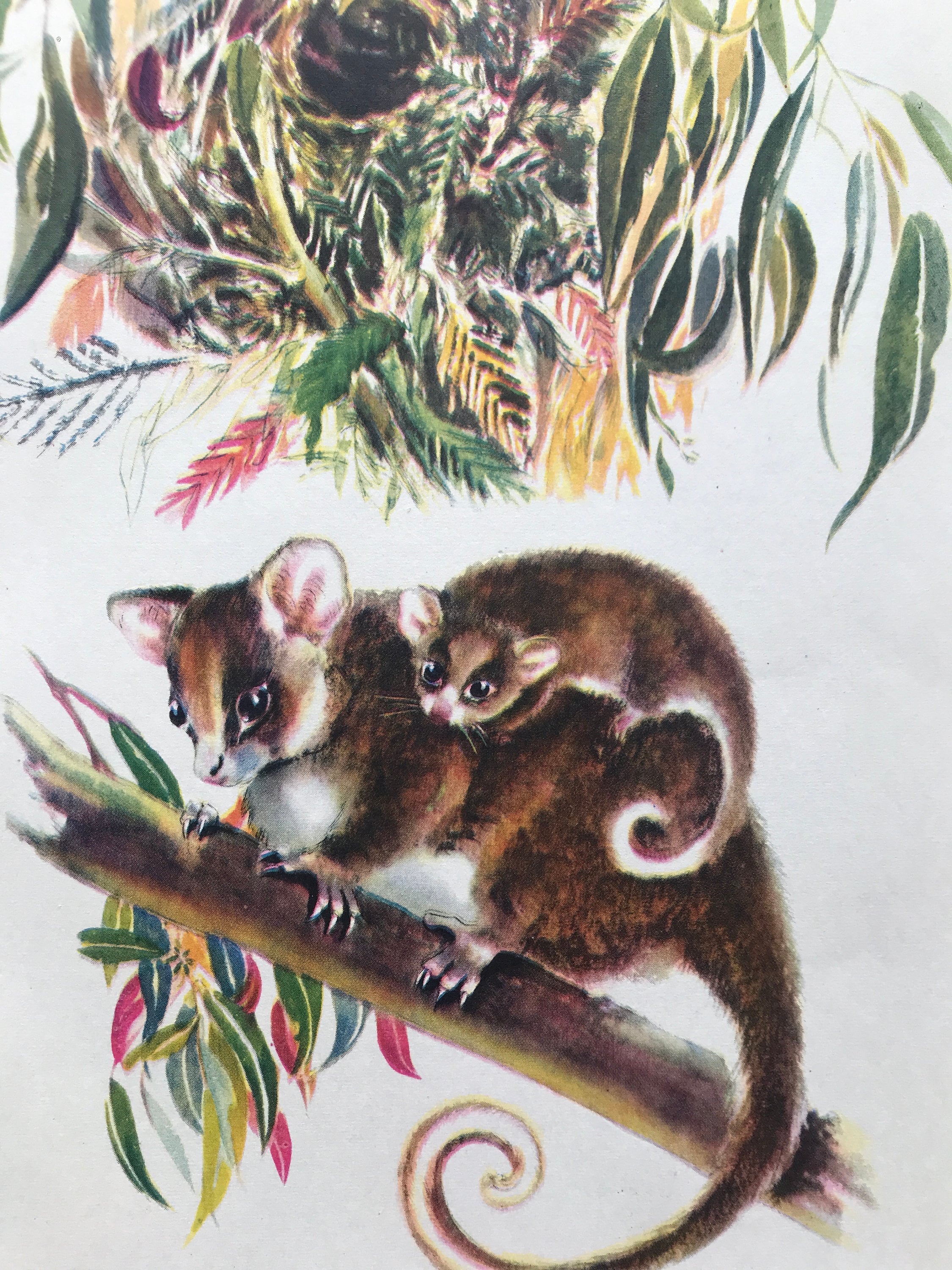This vintage color illustration, reminiscent of the mid-1950s style, features a detailed, hand-drawn portrait of a ring-tailed possum and its baby. The possums are situated on a dark brown tree branch that cuts across the center of the image in a portrait orientation. The adult possum, coated in brown fur with a white underbelly and a pinkish nose, is positioned midway up the image, facing the left. Its large pink ears and strikingly big eyes, which occupy a significant portion of its face, add an engaging expressiveness to its features. The mother possum’s long tail, which curls elegantly at the end, extends toward the bottom right corner of the illustration. Clinging securely to the mother's back, the baby possum mirrors its parent with similar facial characteristics, including larger ears and a distinctive white-tipped tail.

The background showcases a vibrant cross-section of a rainforest with an array of multi-colored leaves—green, yellow, red, orange, pink, blue, and dark purple—mish-mashed at the top and scattered around the tree limb, creating a lively and immersive environment. The meticulous detailing of the fur textures on the possums and the foliage behind them enhances the illustration’s vintage charm, making it both a captivating and nostalgic visual experience.